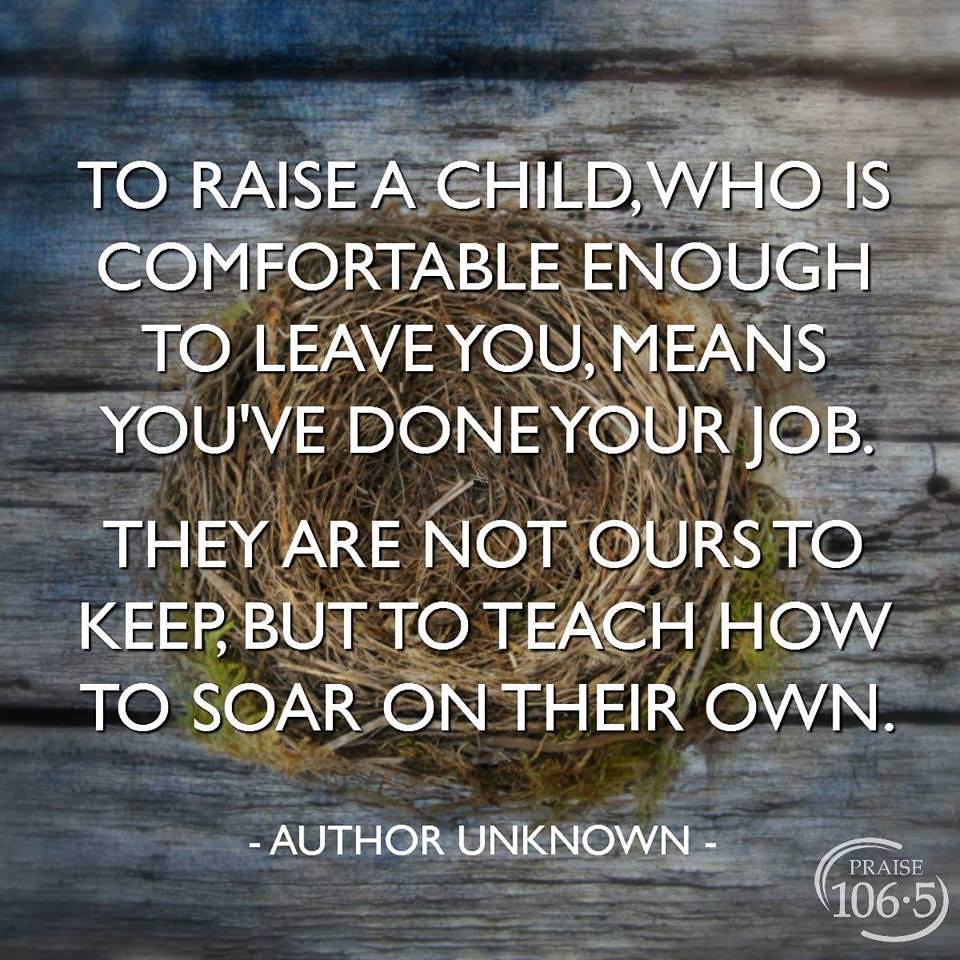This image, reminiscent of an inspirational social media meme, features a well-worn, wooden floor or outdoor patio blurred into shades of dark blue and black at the top. At its center lies a modest bird's nest, crafted from light brown twigs with touches of moss around the edges. Overlaid in white, capitalized letters is an evocative quote: "To raise a child who is comfortable enough to leave you means you've done your job. They are not ours to keep but to teach how to soar on their own." The quote is attributed to "Author unknown," with Praise 106.5 noted in the lower right corner, potentially indicating the post's source. The nest serves as a poignant metaphor, likening children growing up and leaving home to birds leaving the nest, reaching out to parents who are navigating the bittersweet transition of letting their children fly on their own.